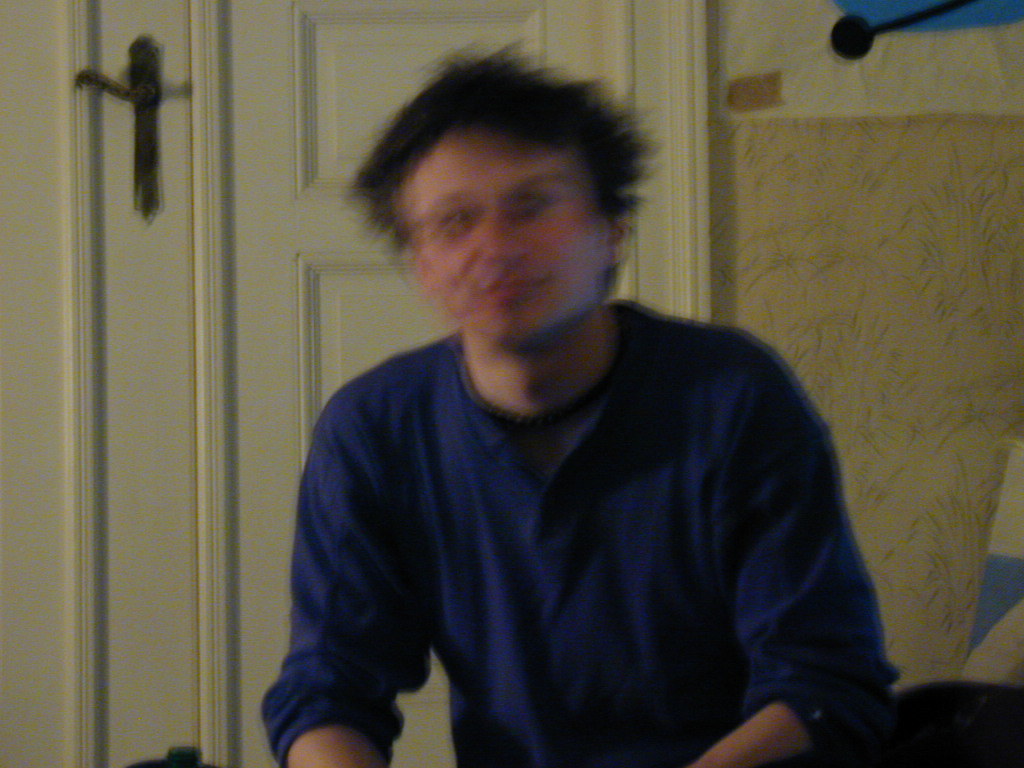The photograph captures a man with short, messy brown hair sitting in front of a skinny white door. The image is notably blurry, causing his face to be obscured with motion blur, although he appears to be smiling. He wears a long-sleeved blue shirt with the sleeves rolled up to his elbows, creating visible wrinkles around the forearms. The door behind him features a black lever handle, and there is a coat rack mounted at the top left. To the right of the image, a wall transitions from white to beige wallpaper adorned with a green and beige floral pattern, accompanied by a blue object partially cut off and a white and cyan checkered item. The man is light-skinned, and the overall image has a lot of blur, affecting the clarity of various details.